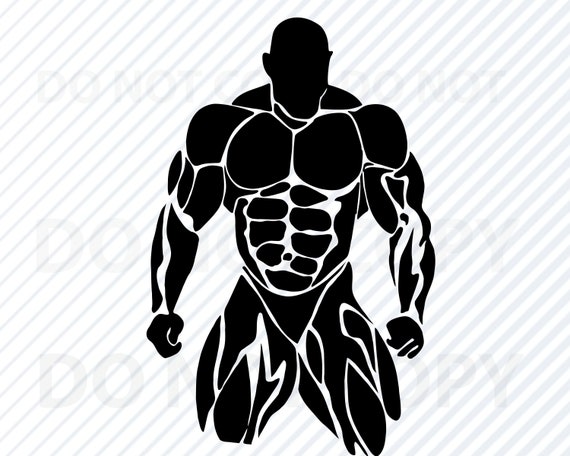This is a detailed drawing of a muscular male figure, presented on a background with light blue diagonal pinstripes running from the lower left to the upper right. The background also features a light gray watermark with the words "do not copy." The figure itself is rendered in black with intricate white outlines that meticulously highlight the muscular anatomy. Each muscle group—including those in the legs, chest, arms, and particularly the well-defined abs—is prominently displayed. Additionally, there are lines on the arms that suggest arteries and veins. The figure's face is a dark silhouette without any facial features, though the white outlines define the chin. He stands with arms straight down, and the drawing simulates the appearance of an eight-pack and the detailed back muscles, typical of a bodybuilder. The lower part of the drawing includes the white-outlined indication of minimal, competition-style underwear, emphasizing the leg muscles.